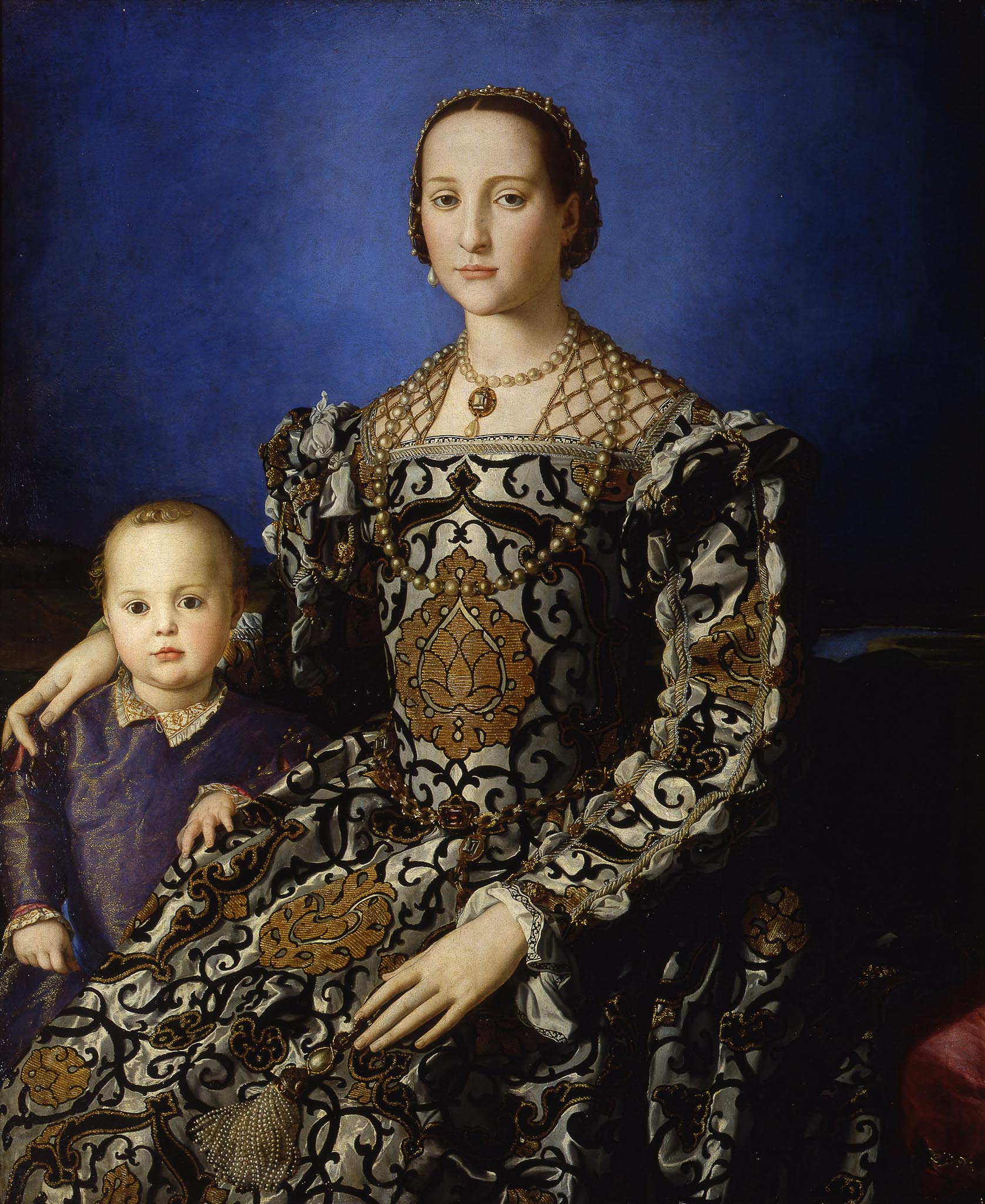The painting captures an elegant scene featuring a woman, prominently positioned at the center, clad in an ornate, long silver-gray dress adorned with intricate black swirls and brown crests. Her porcelain white skin contrasts with her deep brown eyes, and a faint blush touches her cheekbones. Her dark hair is pulled back tightly into a bun, accentuated by a gold headband. Delicate golden strings form a web across her shoulders, securing her dress in place. Around her neck, she wears two necklaces—a choker-length pearl strand and a longer pearl necklace draped to the middle of her chest, possibly with a pendant. One of her hands rests gracefully on her hip while the other tenderly encircles a young boy standing beside her.

The boy, dressed in a dark blue outfit, appears to be around three years old. He has short, light-colored hair and shares his mother's brown eyes and rosy cheeks. One of his hands rests gently on the woman's thigh, while the other hangs by his side. The backdrop of the painting transitions from a soft, light blue behind the woman's head to a darker blue toward the edges.

Both subjects exude a timeless quality, reminiscent of portraits from the 1600s to 1800s, blending historical attire with a detailed, almost computer-generated precision in the oil painting technique.